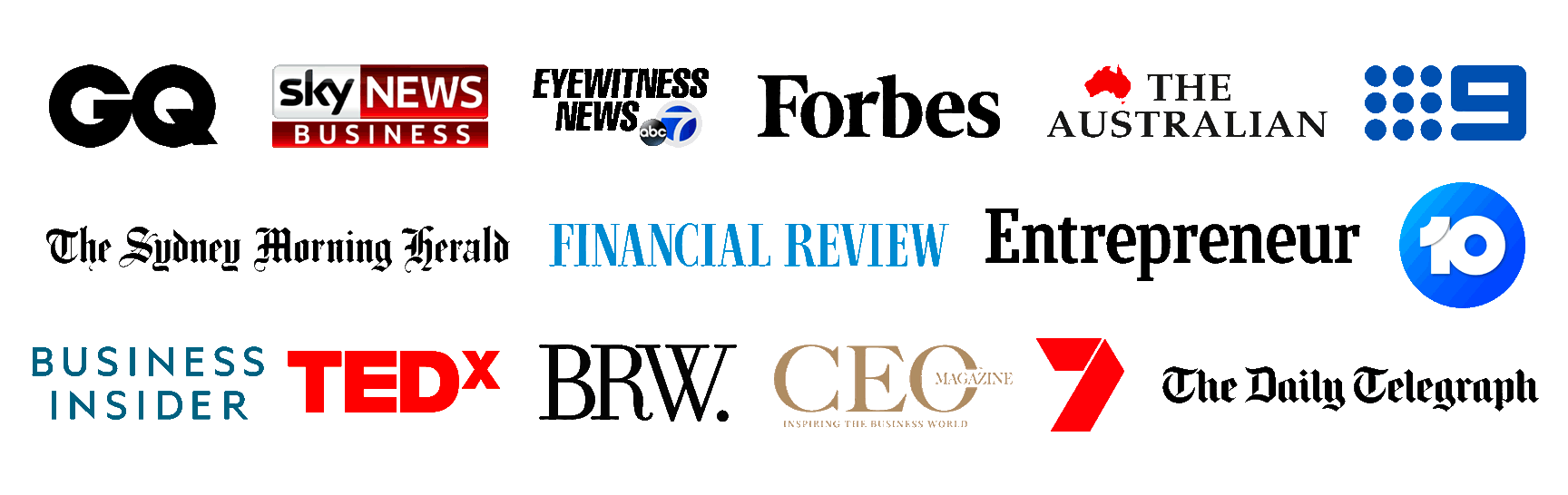This image, captured from a desktop screen, features a visually striking, rectangular poster displaying a mosaic of logos from various media companies, television broadcasters, and magazines. The logos, arranged side by side in three rows, represent a diverse array of prominent Australian and international media brands, each displayed in its original colors. The vibrant assembly includes notable names such as GQ, Sky News Business, Eyewitness News, AB7, Forbes, The Australian, Channel 9, Channel 10, The Daily Telegraph, Channel 7, CEO Magazine, BRW, TEDx, Business Insider, The Sydney Morning Herald, Financial Review, and Entrepreneur. The poster, reminiscent of what you might see at a sponsored event or behind interviews, effectively encapsulates the collaborative media presence, showcasing the visual identities of these influential entities in a unified and cohesive display.